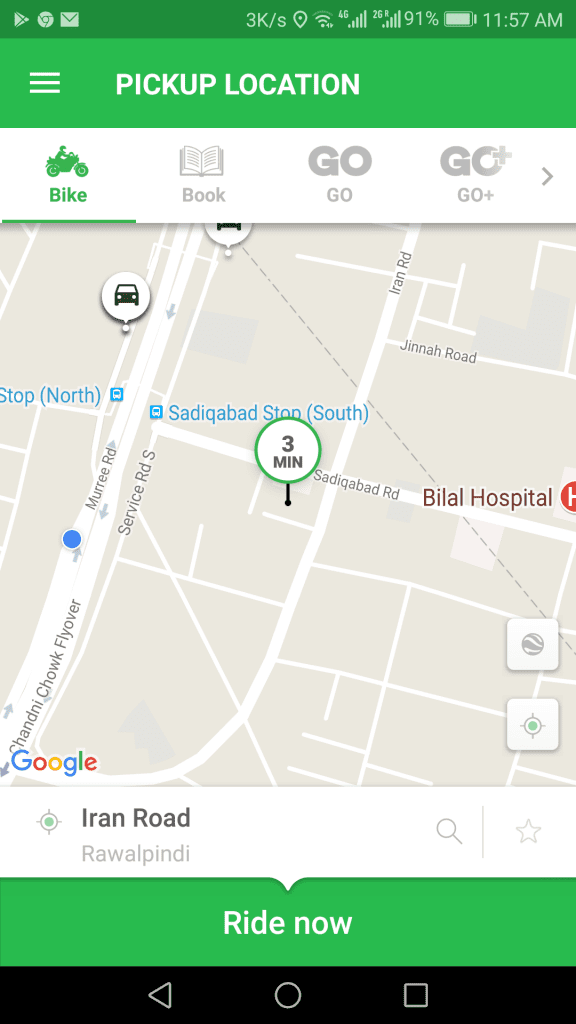This image is a screen capture taken from a digital device displaying a map interface. At the top of the screen, there is a bright green horizontal banner with the text "Pick Up Location" written in white. Below this banner, several selection options are visible. The first option on the left features the word "Bike" alongside a green icon of a bicycle, both underlined in green. Adjacent to it, the next option displays a grayed-out book icon with the word "Book" underneath. The following two options both show the word "GO" in capital letters.

In the lower portion of the screen, the actual map is displayed. It features a light gray background, with roads and intersections highlighted in white. Prominently placed in the center of the map is a white circle outlined in green, labeled "3 minutes." 

On the right side of the map, "Bilal Hospital" is written in dark brown. At the bottom left corner of the map, the text "Iran Road" is visible. The map's visual elements and labels provide clear indications of specific locations and navigation options, catering to a user potentially looking for directions, bookings, or other services related to these areas.